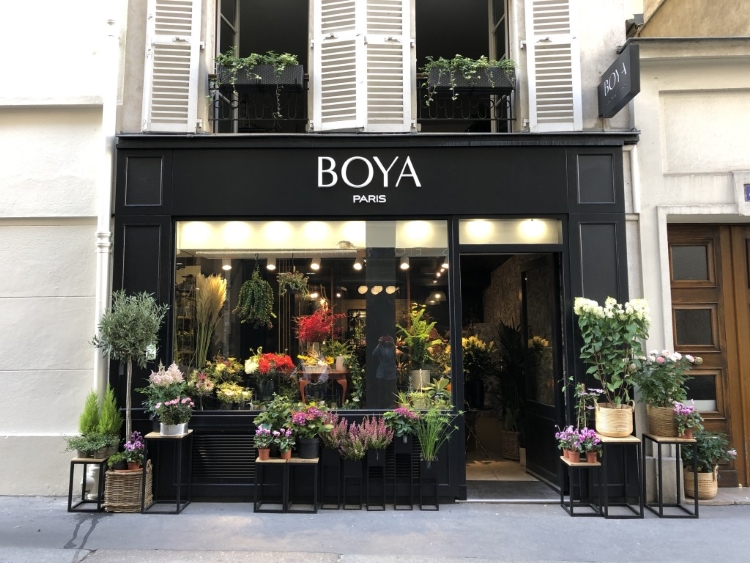The picture showcases a flower shop named "Boya Paris," situated at the center of the image. The storefront is distinctly black, standing out against the surrounding white buildings. The white sign at the top of the shop, designed in clean sans-serif capital letters, prominently reads "BOYA," with "PARIS" in smaller letters underneath. The storefront boasts large glass windows that provide a clear view inside, where bright circular lights illuminate an array of flowers and plants.

Outside, the shop spills over with vibrant greenery. Numerous black metal tables with white tops are adorned with flower pots and planters filled with a variety of plants and flowers, ranging in colors from reds and purples to pinks, whites, and yellows. Among these are tall decorative leaves, ferns, large bushy plants with white blossoms, and topiary arrangements. 

The open doors invite customers into a welcoming space while additional flowering plants are arranged to the right of the entrance. Above the shop, two windows with open white wooden shutters reveal dark interiors but are complemented by black window boxes overflowing with cascading ivy and vine plants. To the right, there's a white adjoining building featuring a brown wooden door and two whitened windows with flower pots, adding a quaint touch to the picturesque street view.